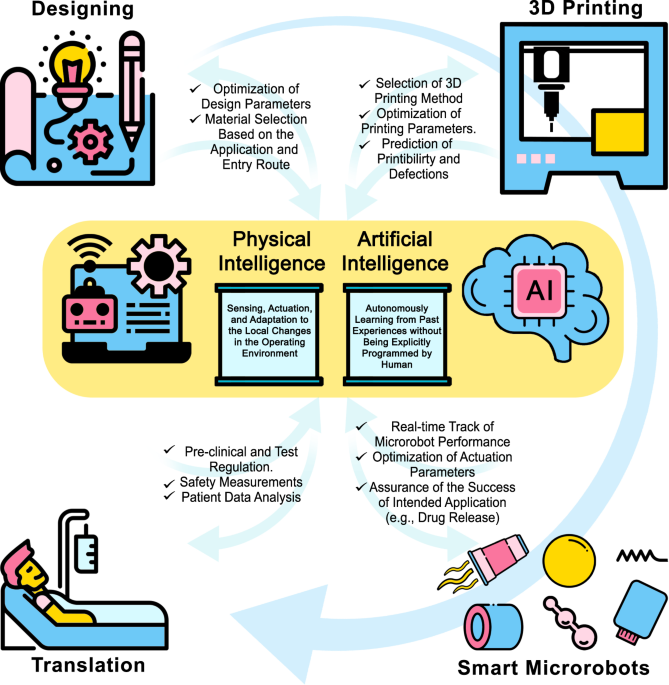This detailed infographic illustrates a cyclical process with four interconnected stages—Designing, 3D Printing, Smart Micro Robots, and Translation—all converging into a central concept of physical and artificial intelligence. 

In the top left, "Designing" is represented by an image of a blueprint, a light bulb, a gear, and a pencil, highlighting the optimization of design parameters and material selection based on application and entry route. The top right corner features a diagram of a 3D printer, focusing on the selection of 3D printing methods, optimization of printing parameters, and prediction of printability and defections.

In the bottom right, "Smart Micro Robots" is depicted through ambiguous shapes like a sphere and interconnected bubbles, emphasizing real-time tracking of micro-robot performance, optimization of actuation parameters, and assurance of successful application, exemplified by drug release. The bottom left illustrates "Translation" with an image of a person in a hospital bed hooked up to an IV, detailing preclinical and test regulations, safety measurements, and patient data analysis.

All these quadrants are linked by a cyclic arrow and feed into a central bubble labeled "Physical Intelligence," which includes a representation of a computer with a gear and a robot with a Wi-Fi symbol. This central concept focuses on sensing, actuation, and adaptation to local changes in the operating environment. Additionally, "Artificial Intelligence" is depicted with a brain and the letters AI, highlighting autonomous learning from past experiences without explicit human programming. The overall theme suggests the application of advanced 3D printing technology in medicine, driven by intelligent systems capable of optimizing and adapting based on real-time data and historical learning.